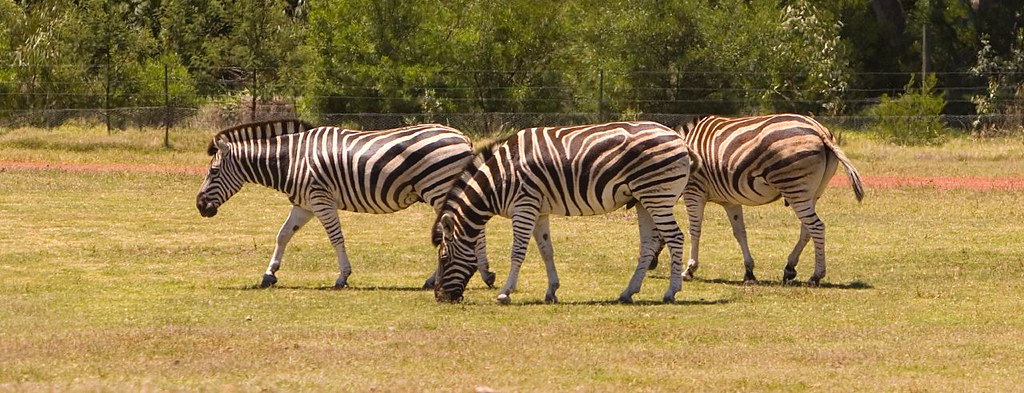This color landscape photograph captures a serene scene of three zebras on a light green, low-cut grassy field, dotted with occasional brown patches near the bottom of the image. The expansive field, which resembles a well-maintained but unnatural environment, is bordered by a thin wire fence supported by black wooden poles. Beyond the fence, a dense array of green-leafed trees forms a vibrant backdrop. The three zebras are all oriented towards the left side of the image: the one in the back appears to be walking, the middle one is grazing with its head down, and the rightmost zebra is angled slightly away from the viewer, with its head obscured behind the grazing zebra. The overall composition emphasizes the peaceful coexistence of these animals within a managed, yet picturesque setting.